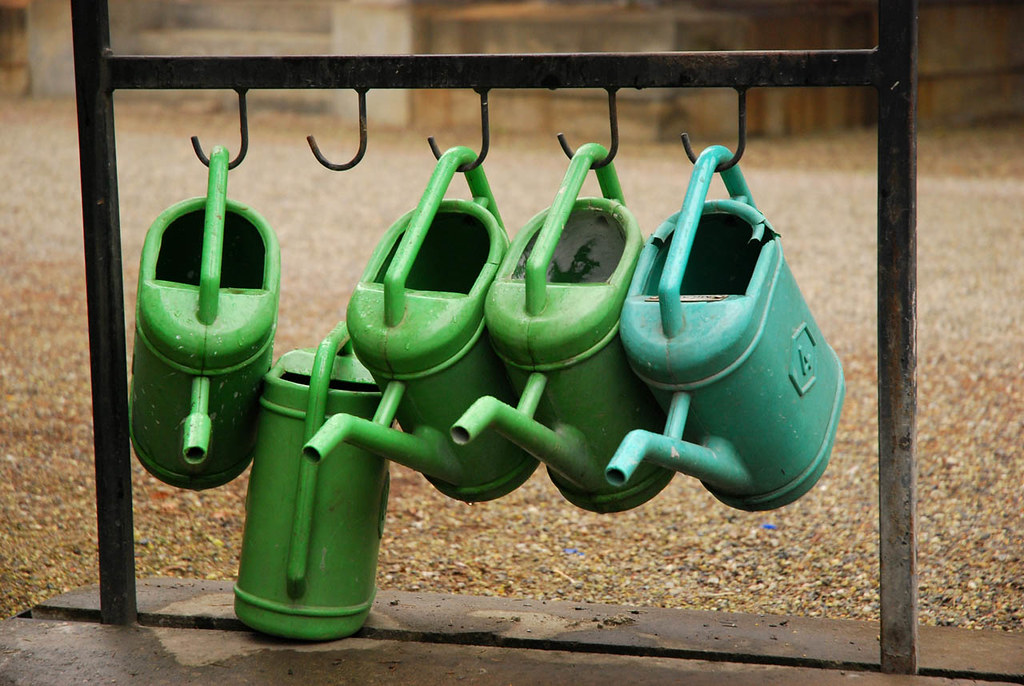An outdoor photograph showcasing five weathered metal watering cans. Four of these cans—three green and one blue—dangle from J-shaped hooks on a black iron stand in the shape of an 'H'. Notably, the blue watering can bears the number "4" and shows signs of wear around the rim. The green watering cans, slightly wet with droplets visible, hang with their spouts facing the viewer. On the ground, between the hanging cans, another green watering can rests facing away. The iron stand exhibits some rust and is anchored in a base that seems to be a combination of wood and metal, partially obscured. The background features a tan and gray gravel surface and hints of a wooden structure in the distance, suggesting this setup might be in a community garden.